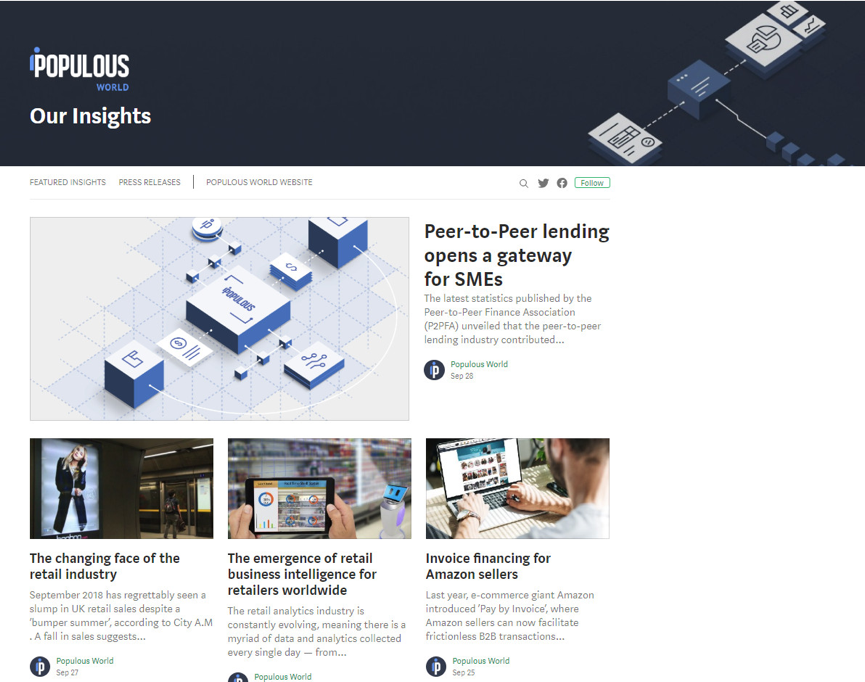This is a screenshot of a website featuring a navy blue banner at the top with light blue graphic elements. The banner displays the words “Populous” in white, “World” in blue, and “Insights” in green. Beneath this banner is a blue and white computer graphic accompanying a headline that reads, “Peer-to-Peer Lending Opens a Gateway for SMEs.” Below this headline, there is a section with three separate articles:

1. The first article features an image of a woman and is titled "The Changing Face of the Retail Industry."
2. The second article shows an individual holding a tablet and is titled "The Emergence of Retail Business Intelligence for Retailers Worldwide."
3. The third article is titled "Invoice Financing for Amazon Sellers."

Each article is timestamped and the source is attributed to “Populous World,” which is highlighted in green.